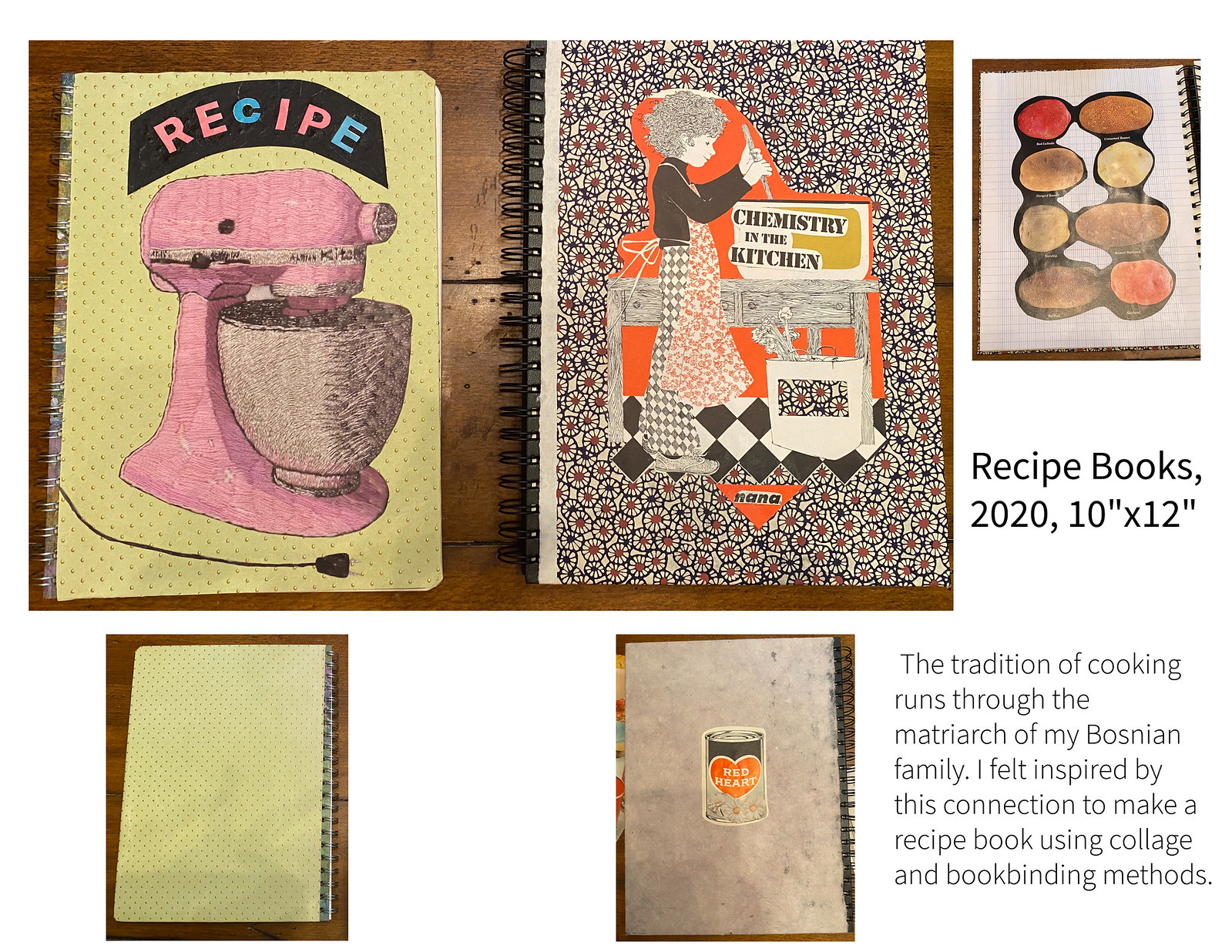In the upper right corner, the largest image displays two spiral-bound notebooks resting on a wooden table. The left notebook features a yellow cover with a black banner that spells "Recipe" in pink and blue letters, accompanied by an illustration of a pink stand mixer. Adjacent to it, a notebook with a daisy-patterned cover titled "Chemistry in the Kitchen" showcases a vintage-style drawing of a woman in an apron, possibly labeled "Nana," mixing ingredients at a wooden table. Another spiral notebook with a collage of magazine pictures—possibly stones or eggs—is visible to the right of this.

In the lower section, the back covers of the two notebooks are shown. The yellow recipe book continues the spiral binding design, while the back of the "Chemistry in the Kitchen" book features an illustration of a can labeled "Red Heart" with a matching red heart icon. Next to these, the text reads "Recipe Books 2020, 10 inch by 12 inch." Additional text captures the creator's inspiration, "The tradition of cooking runs through the matriarch of my Bosnian family. I felt inspired by this connection to make a recipe book using collage and bookbinding methods," underscoring the sentimental and artistic drive behind these cookbooks. The overall presentation reflects a scrapbook aesthetic, blending vibrant colors and thoughtful collages to celebrate family and culinary traditions.